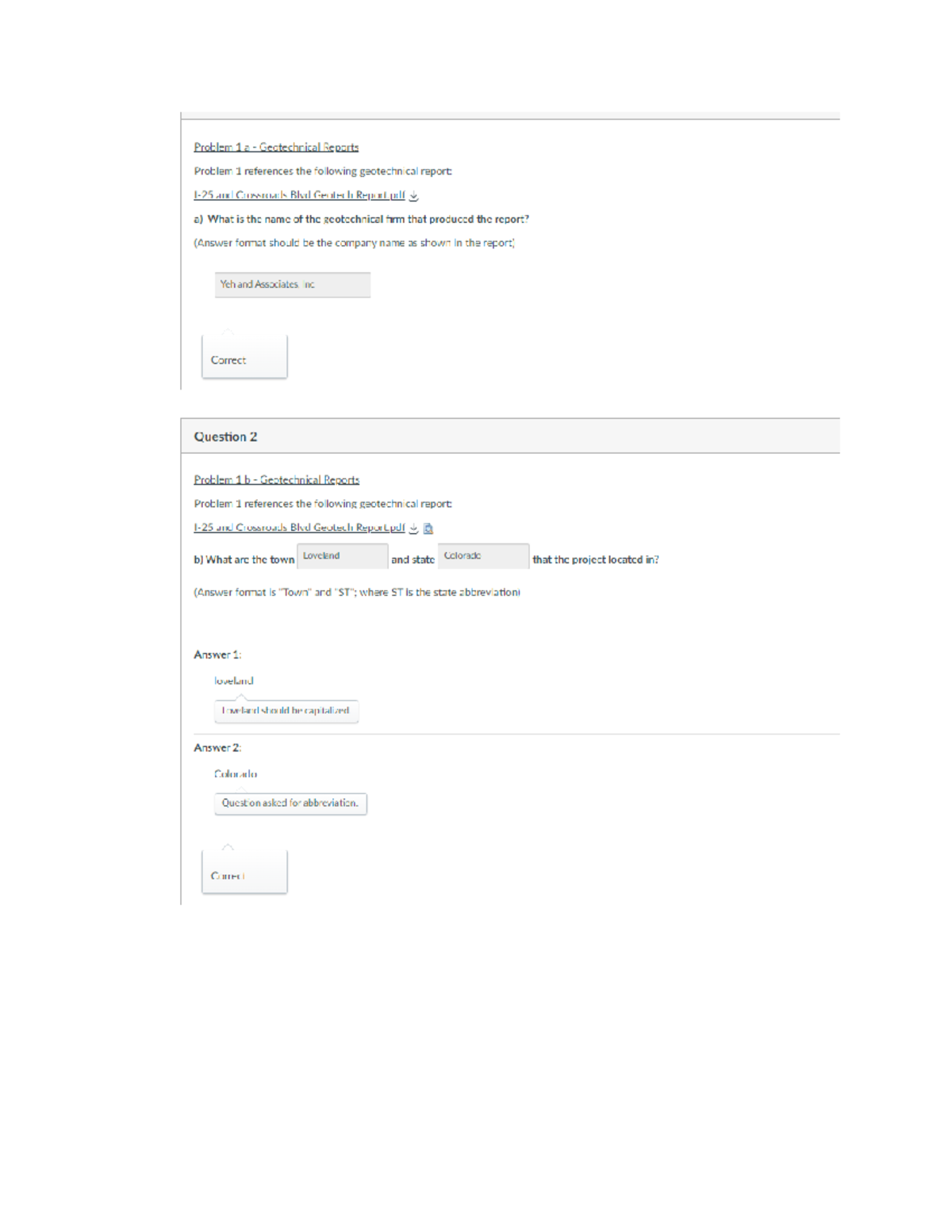**Detailed Caption:**

The screenshot displays two stacked boxes, each containing sections of a form with information and questions related to geotechnical reports, both set against a white background.

**Top Box:**
- Title: "Problem 1A - Geotechnical Reports"
- Text: "Problem 1 references the following geotechnical report:"
  - Information:
    - "I-25 and Crossroads Boulevard, geotechreport.pdf" (associated with a download symbol)
  - Question (labeled "A)"): "What is the name of the geotechnical firm that produced the report?" (Note: "Answer Format should be the company name as shown in the report.")
  - Response Box (filled in): "YEH and Associates, Inc." 
  - Feedback: "Correct" in a box underneath the answer.

**Bottom Box:**
- Title: "Question 2"
  - Subtitle: "Problem 1B - Geotechnical Reports"
  - Text: "Problem 1 references the following geotechnical report:"
    - Information:
      - "I-25 and Crossroads Boulevard, geotechreport.pdf" (with a download icon and an additional icon resembling a page)
    - Question (labeled "B)"): "What are the town and state that the project is located in?" (Note: "Answer Format is 'Town' and 'ST', where ST is the State Abbreviation.")
    - Response:
      - Town: "Loveland" (properly capitalized)
      - State: "Colorado" (not abbreviated)
    - Feedback:
      - Instruction: "Loveland should be capitalized."
      - Instruction: "The question asked for the state abbreviation."
      - Verification: "Correct" in a box under each response.

In essence, the screenshot captures the process of verifying the accuracy of answers pertaining to the identification of a geotechnical firm and the location details of a project, highlighting requirements for correct formatting and capitalization.